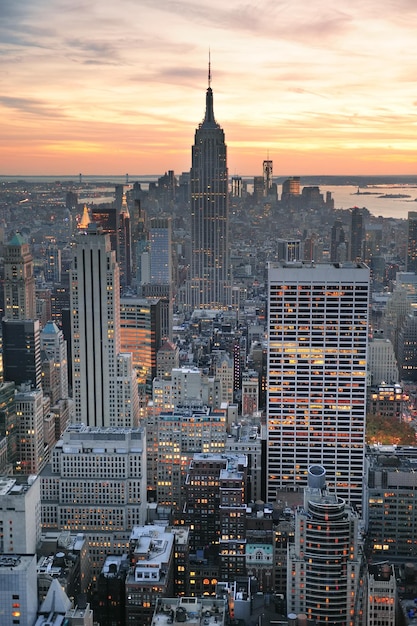This striking photograph captures an iconic view of downtown Manhattan, centered on the majestic Empire State Building with its pointy top rising prominently among a sea of gray skyscrapers. Taken from a high vantage point, the image provides a sweeping perspective over the city, revealing an array of other tall buildings bathed in the soft glow of early evening lights. The sky is a mesmerizing blend of orange and peach hues near the horizon, gradually deepening to a blue and purple gradient towards the top, indicating the sun has just set. Some windows in the buildings are lit with warm yellow tones, contrasting with the cool, muted colors of the surrounding structures. In the distance, the Statue of Liberty can be seen to the upper right, and the reflection of the sky's colors shimmers on the water at the edge of the city, adding to the scene’s depth and serenity.